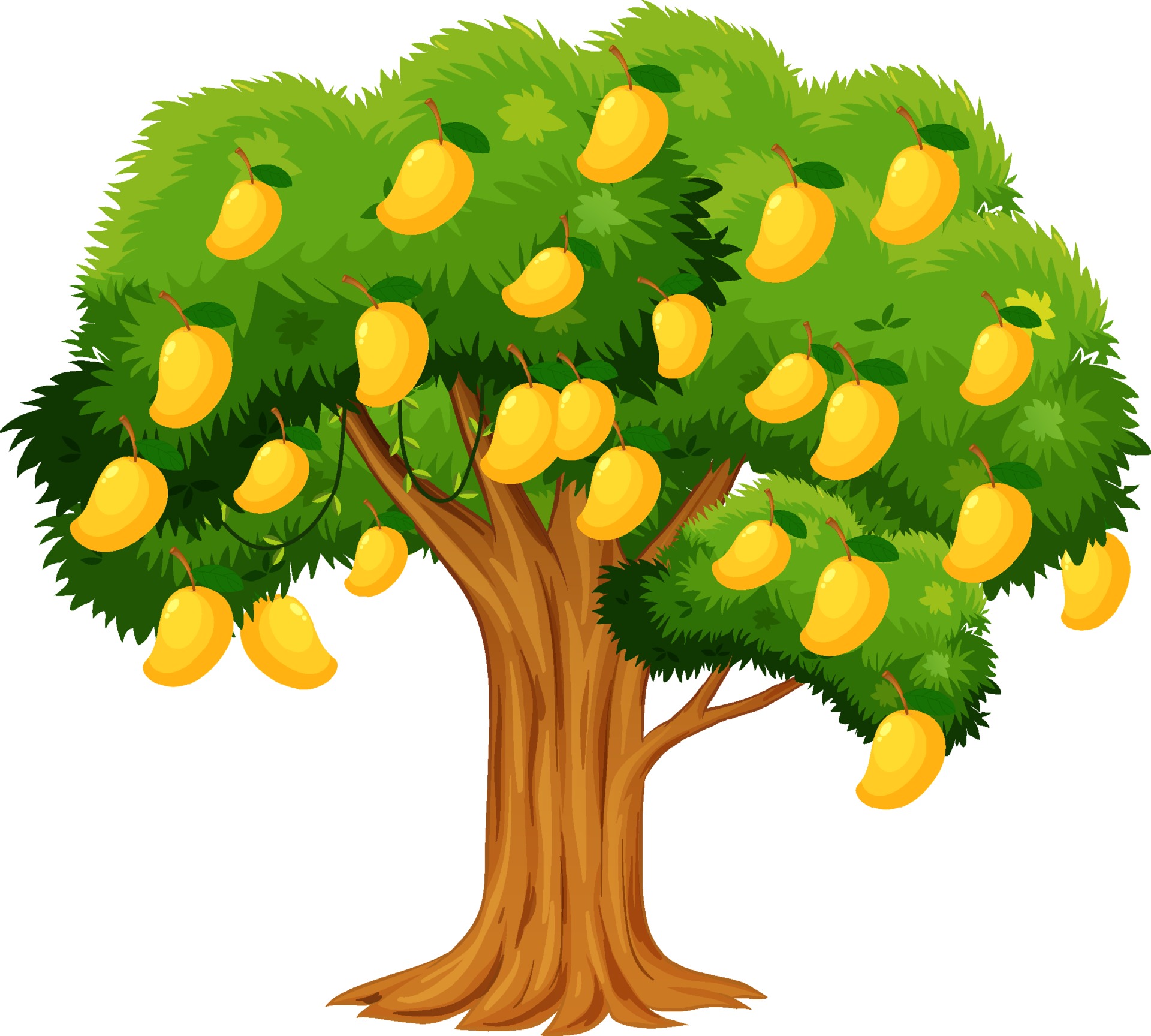This digital illustration features a vibrant mango tree set against a stark white background. The tree boasts a thick, ridged trunk shaded in varying tones of light to dark brown. The branches are densely adorned with leaves that are predominantly light green, interspersed with some darker green foliage. Dangling from the branches are approximately 26 large, oval-shaped mangoes, transitioning in color from yellow to orange, giving a realistic depiction of their ripening process. These mangoes are fairly uniform in shape, resembling jellybeans. The entire scene is presented with vivid colors, highlighting the tree's lush greenery and the golden-yellow to orange mangoes, creating a visually striking digital artwork.